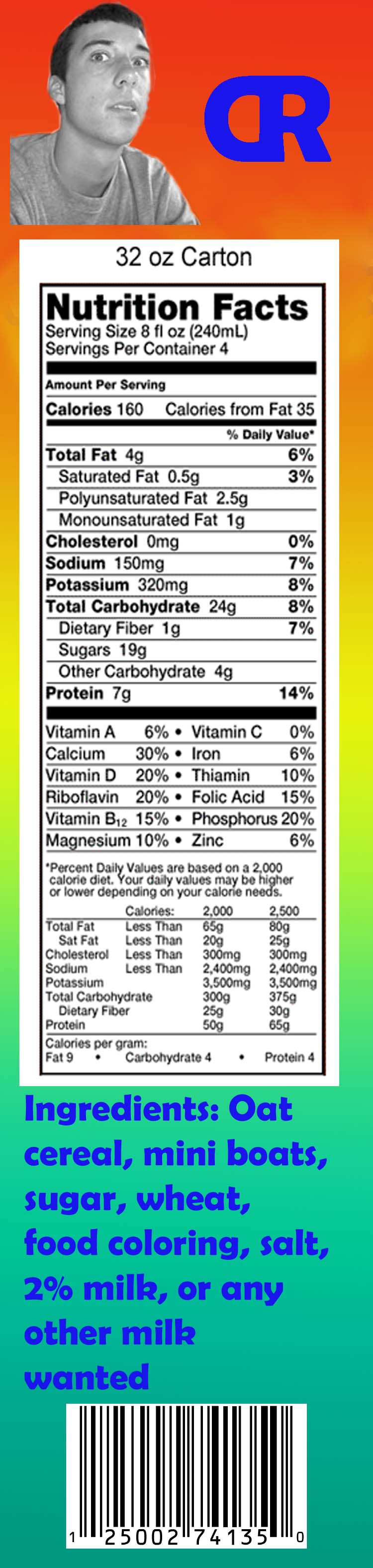The image showcases a nutrition label set against a rainbow-colored background transitioning vertically from red to blue. At the top of the image is a picture of a young man with very short hair, displaying his head and upper chest, who is looking directly at the camera. Beside him are the letters "CR" in large, connected blue font. Below this is a detailed nutrition label for a 32-ounce carton of an unspecified product, listing the serving size as 8 fluid ounces with 4 servings per container. The nutritional information includes calories (163), calories from fat (36), and other standard nutritional details. Underneath the nutrition label is an ingredient list stating oats, cereal (mini boats), sugar, wheat, food coloring, salt, 2% milk, or any other preferred milk. This ingredient list is written in a bright blue color and appears to be digitally altered. At the very bottom, there is a white rectangle containing a barcode with the number series 125002741350. The overall composition and some elements, such as the ingredient list and the rainbow background, give the image an artificially edited appearance.